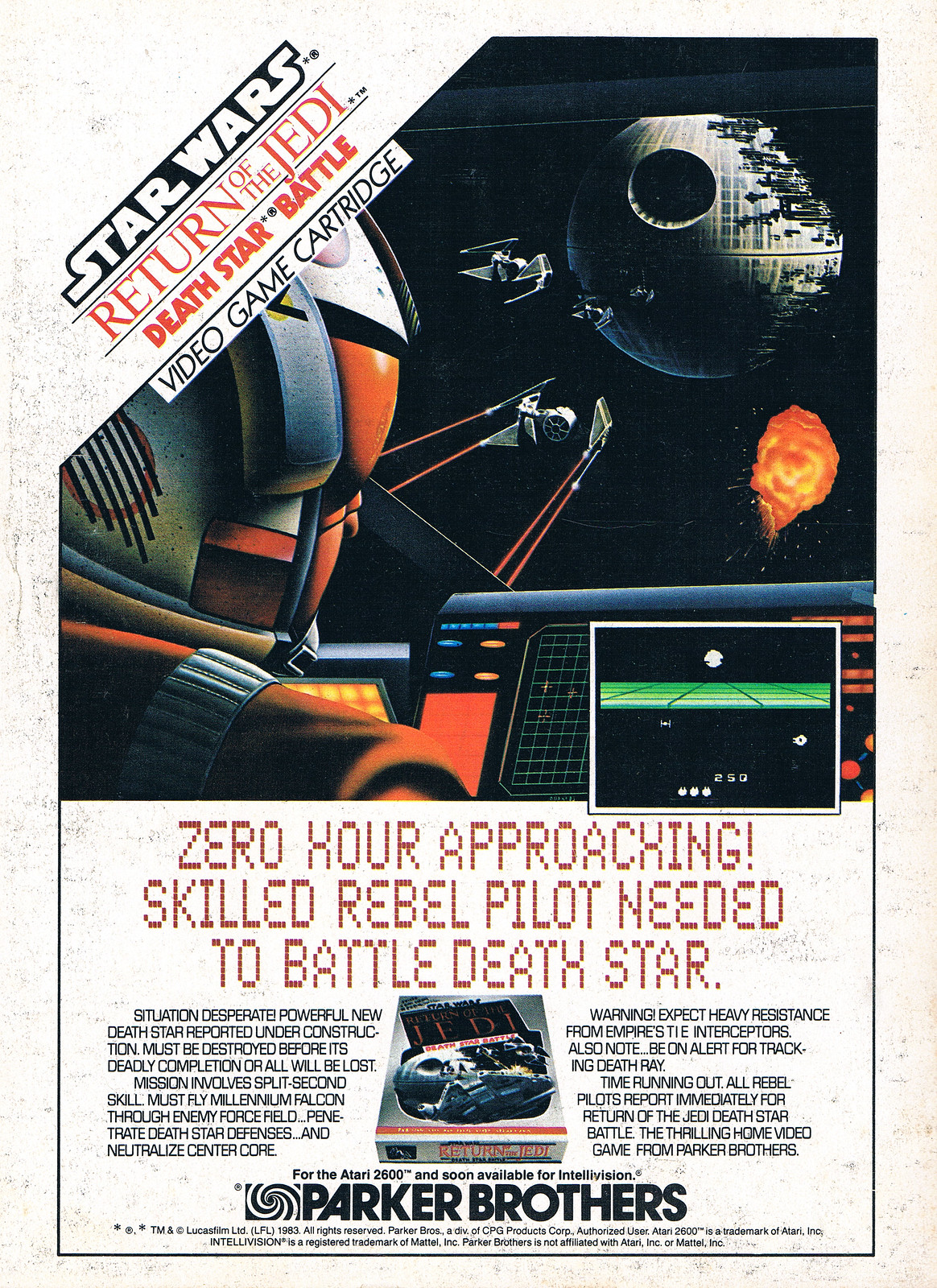This is a full-page advertisement for the Star Wars Return of the Jedi Death Star Battle video game cartridge by Parker Brothers, designed for the Atari 2600 and soon available for Intellivision. The ad features a cream-colored background and prominently showcases the game's title in a triangle cutout positioned at a 45-degree angle in the top left corner. The focal point of the design is a cutoff black square image displaying vivid concept art from the movie, with an orange and white spaceship, the Millennium Falcon, navigating against the backdrop of the iconic Death Star in outer space. Below the visual, red-lettered text on a white background urgently states: "Zero Hour Approaching. Skilled Rebel Pilot Needed to Battle Death Star. Situation Desperate. Powerful new Death Star reported under construction. Must be destroyed before its deadly completion or all will be lost." Further details explain the mission requirements, emphasizing quick reflexes to pilot the Millennium Falcon through enemy force fields, penetrate the Death Star's defenses, and neutralize its center core, all while facing heavy resistance from the Empire's TIE interceptors and a tracking death ray. Additional descriptions at the bottom highlight the thrilling nature of the game, calling all rebel pilots to report immediately. The Parker Brothers logo is boldly displayed at the bottom, making it clear that this engaging video game experience is brought to you by a well-known name in gaming.